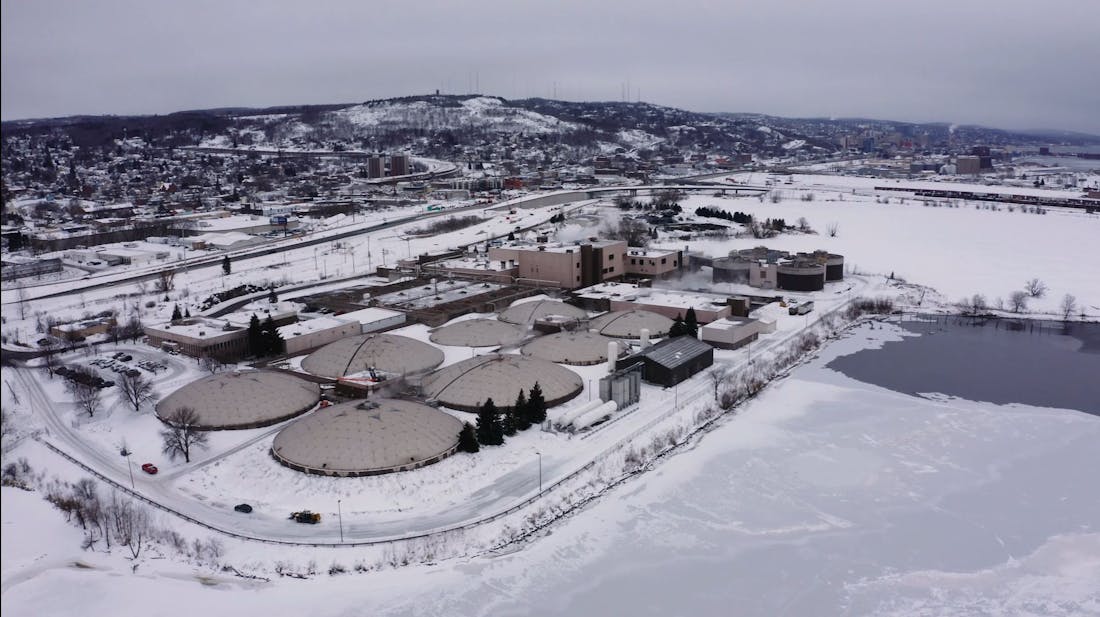This image presents a serene, snow-covered, small town captured from a bird's eye view. The sky is a muted gray, emphasizing the winter setting and casting a calm stillness over the scene. A prominent feature of the landscape is a hill or large snow-covered rise in the background. In the middle right side of the image, there is a partially frozen river or lake, the thawed water contrasting with the icy expanse around it. The town features an array of bland, beige buildings, including several dome structures, nestled among some snow-dusted pine trees. The roads are partially covered in snow, with a few parked cars visible, adding to the tranquil and undisturbed atmosphere. No people are present in the image and there is no text to read, leaving the viewer to absorb the quiet and somewhat bland yet peaceful wintery environment. The scene's landmarks and structures are lightly detailed, providing a modest yet picturesque glimpse of the town in the cold season.